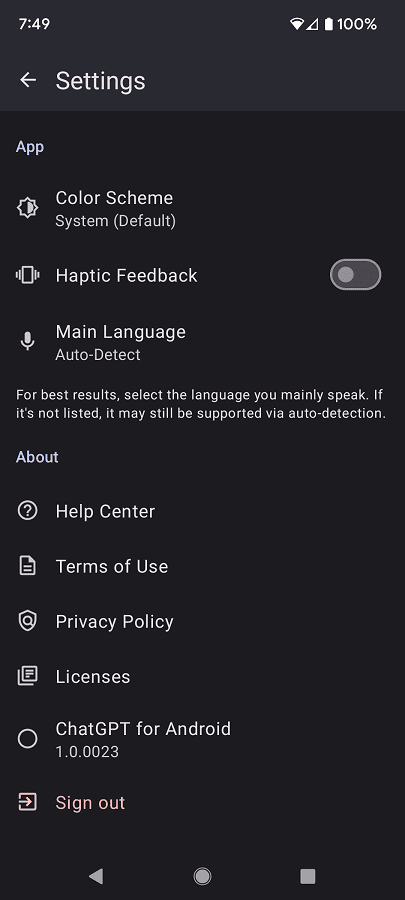The image depicts a screenshot from a mobile device, likely a smartphone or tablet, due to its long and narrow rectangular aspect ratio. At the top of the screen, the time is displayed as 7:49, and the device shows a full battery at 100% with visible wireless signal indicators. The overall theme is predominantly black, with the text in white or gray, indicating a dark mode setting.

The upper section of the image includes the Settings menu, which is labeled as "App Settings.” Below this header is a back arrow icon. Underneath, there are three options: "Color Scheme," "Haptic Feedback," and "Main Language," each accompanied by an icon. To the right of these options are toggle buttons, which appear grayed out, suggesting they are disabled.

Beneath these settings, there is a note advising users to select the language they mainly speak for optimal results. It further mentions that if the language is not listed, it might still be supported via auto-detection.

Scrolling further down, the screen shows an "About" section with the following entries: "Help Center," "Terms of Use," "Privacy Policy," "Licenses," "Check GPT for Android," and a "Sign Out" button, which is highlighted in a pinkish hue. Each of these entries is also accompanied by an icon. 

Finally, at the bottom of the screen, three icons commonly found on Android devices are visible: one for returning to the previous screen, one for going to the home screen, and one for accessing open apps or pages.